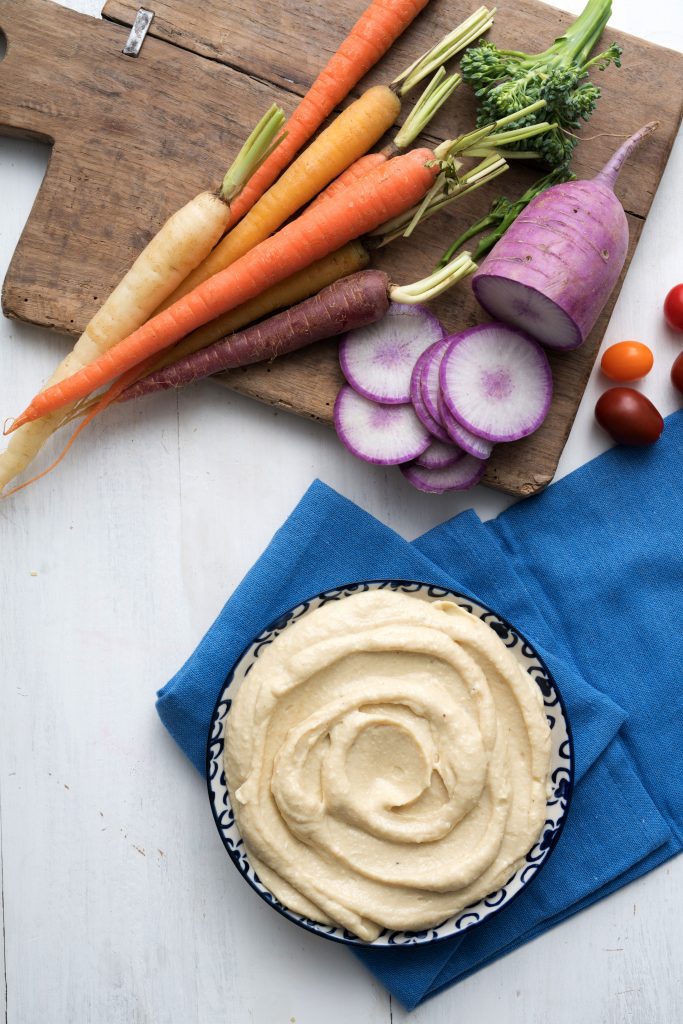This vertical portrait-style photograph captures an assortment of fresh vegetables meticulously arranged on an old-fashioned, well-used wooden cutting board placed on a white wood table. At the heart of the image, the cutting board is adorned with carrots in various hues - dark orange, purple, and white - laid diagonally from the bottom left to the top right, with their green tops still intact. Nestled among the carrots is a small broccoli crown and a collection of thinly sliced pieces of what appears to be a purple parsnip or a large radish. Flanking the right side of the cutting board are small, vibrant grape tomatoes. Below the cutting board lies a white ceramic bowl with an intricate black pattern, filled with a white spread resembling hummus. The bowl is set upon a neatly folded blue knit napkin, completing the rustic and inviting presentation.